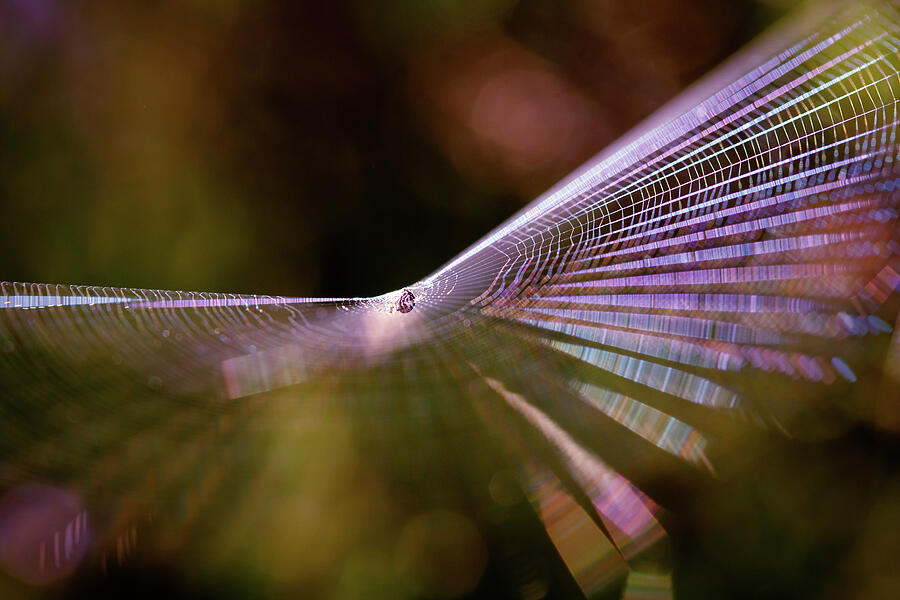The image depicts an extreme close-up, or macro shot, of a small spider positioned centrally in its web. The photograph is highly magnified, showcasing the intricate strands of the spider's web in sharp focus, while the background remains an abstract blur of green shades with focal spots. The web's strands are illuminated in such a way that they appear to be purple and blue, giving the image a surreal, almost futuristic quality. Although the majority of the image is out of focus, creating a hazy, dynamic backdrop of multicolored hues, the clear intricacy of the spider's web stands out as the primary subject amidst the ethereal surroundings.